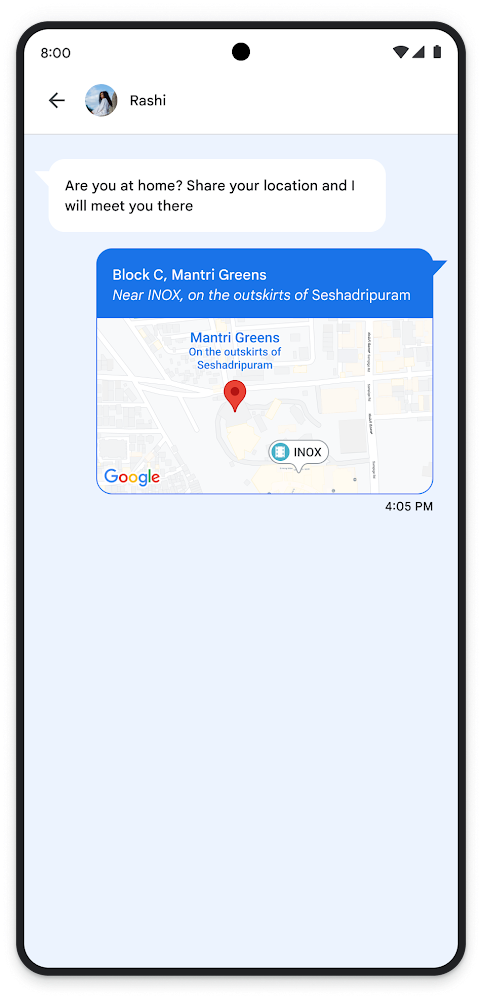In this detailed screenshot captured on a smartphone, the top left corner displays the time as 8:00. In the top right corner, indicators show the phone's battery level, signal strength, and Wi-Fi connection status. The messaging app shows a conversation with a user named Rocky, whose profile icon is visible. Rocky has sent a text saying, "Are you at home? Share your location and I will meet you there." Below his message, Rocky suggests meeting between 4 and 5 p.m. and provides a location: Block C, Manchurian Greens, near Enos, on the outskirts of San Antonio. 

The screenshot highlights a pop-up box from Google Maps featuring a map pinpointing the specified location. This map is depicted with light blue hues, while the pop-up box itself is shaded in a royal blue. A red pin clearly marks the location on the map, providing a vivid contrast against the map's backdrop. The overall visual presentation is both informative and visually structured, offering a clear representation of the suggested meeting arrangement.